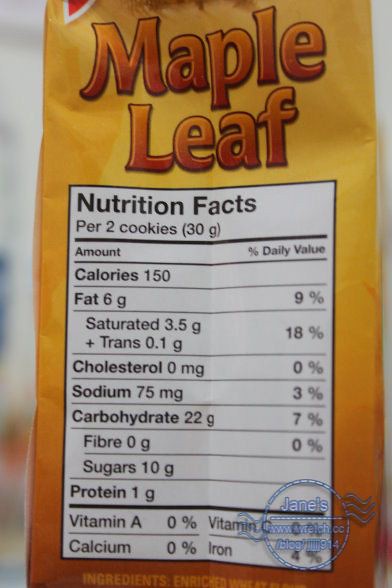This image is a close-up vertical portrait of a nutrition label from a box of cookies named "Maple Leaf". The box features a gradient color scheme, transitioning from darker orange at the bottom to a lighter yellow-orange at the top. The name "Maple Leaf" is prominently displayed in shaded orange letters above the nutrition facts. The nutritional information is presented in a white rectangular box with a black border. The details it includes are per 2 cookies (30 grams): 150 calories, 6 grams of fat (9% DV), including 3.5 grams of saturated fat and 0.1 grams of trans fat, 0 milligrams of cholesterol, 75 milligrams of sodium (3% DV), 22 grams of carbohydrates (7% DV) with 0 grams of fiber, 10 grams of sugars, and 1 gram of protein. Additionally, there are 0% Daily Values for Vitamin A, Calcium, and Vitamin C, and a 4% Daily Value for iron. In the bottom right-hand corner, there is a blurred watermark that reads "Jane's", and part of an address link that is too unclear to make out fully.